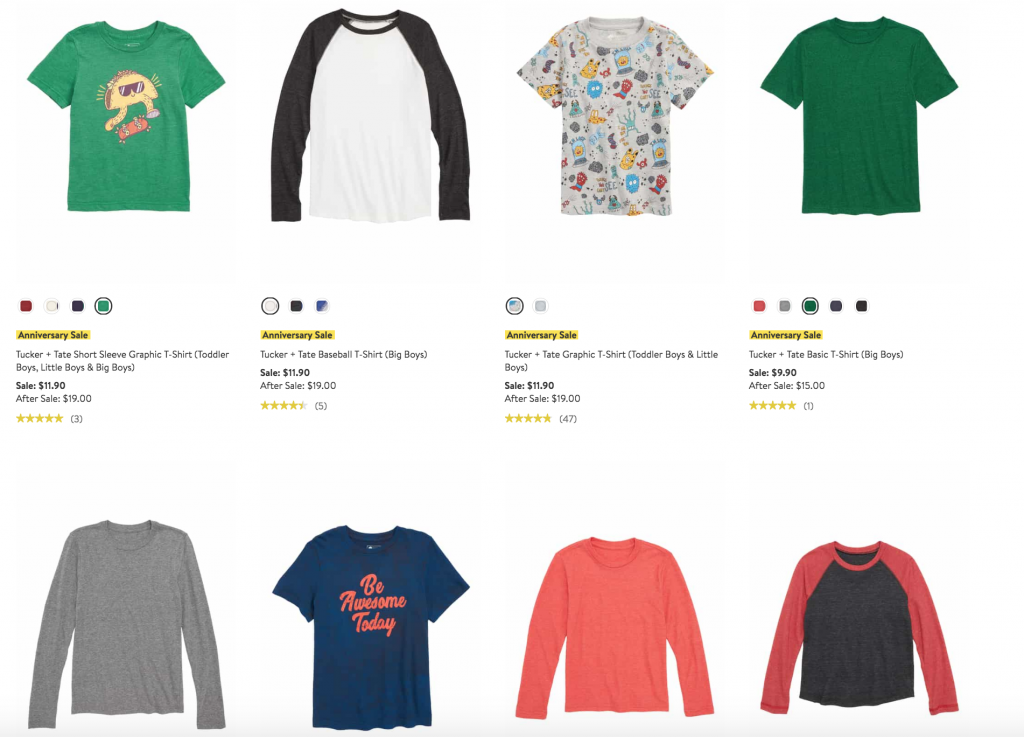This image showcases a variety of boys' t-shirts, both graphic and non-graphic, arranged in two rows. At the top of the page, the first t-shirt is a vibrant green Tucker + T short-sleeved graphic tee featuring a dancing taco, priced at $11.90. Next to it is a white and black long-sleeved Tucker Tate baseball t-shirt for big boys, also at $11.90. The third top-row shirt is a Tucker Tate graphic tee for toddler boys and girls, adorned with small critters on the front, offered at $11.90. The fourth top-row item is an emerald green Tucker Tate basic t-shirt for big boys, priced at $9.90.

On the second row, starting from the left, the first shirt is a long-sleeved gray t-shirt. To its right is a dark blue graphic t-shirt with the inspirational message "Be Awesome Today." The third shirt on the bottom row is a long-sleeved t-shirt in a warm salmon color. The final item in the row is a baseball-style long-sleeved t-shirt featuring a gray body and red sleeves.